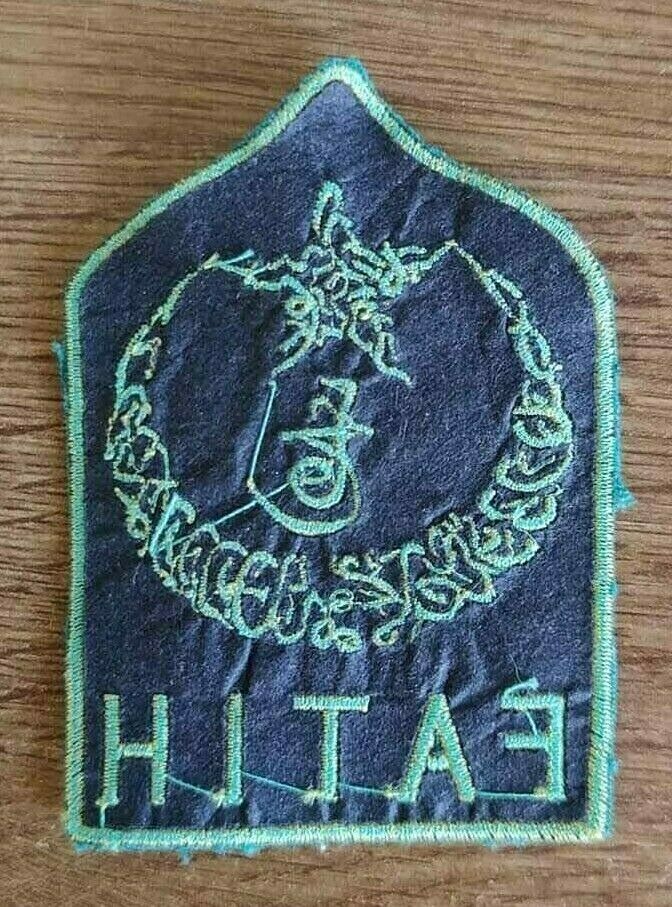The image is a color photograph in portrait orientation, depicting an embroidered patch placed on a medium brown wood-grain table. The patch is rectangular with straight sides and bottom, while the top is curved and pointed, reminiscent of a badge shape. The fabric of the patch is dark blue denim, bordered by a fringe of light minty green stitching. The central design features light green swirly embroidery forming a circular pattern, which surrounds text written in Arabic. Below the circle, the letters "H-I-T-A-F" are visible, although they appear reversed, likely indicating that the patch is shown from its underside, with threads visible suggesting the front would display "F-A-T-I-H". The patch seems best suited for being ironed onto a coat jacket's shoulder area. The photographic style is realism, capturing the intricate details and texture of the embroidery vividly.